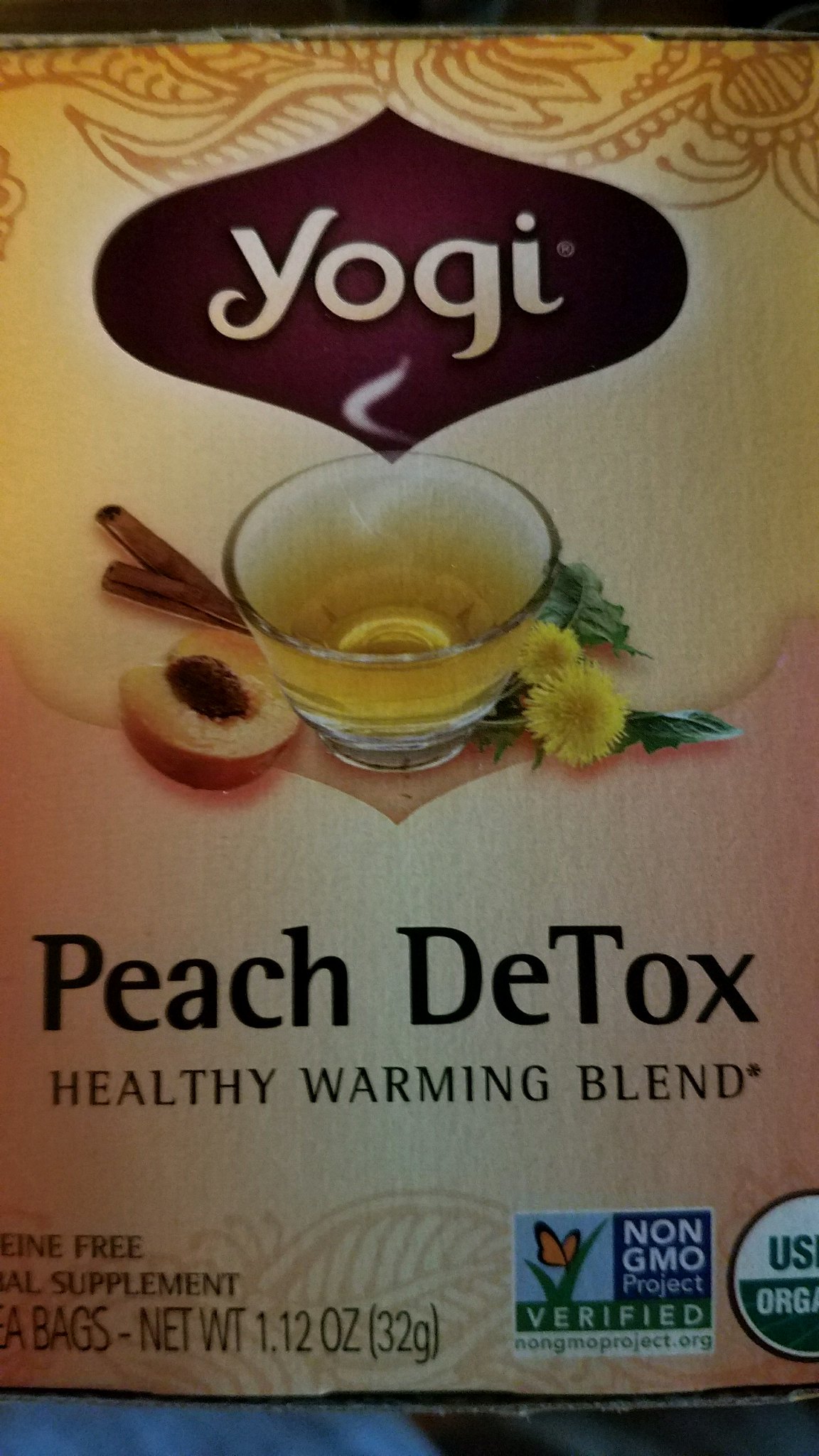This close-up image captures the front label of a Yogi tea box. At the top, in a burgundy teardrop-shape, the brand name "Yogi" is prominently displayed. Below it, a small glass cup contains steaming, yellowish tea, accompanied by a peach slice and some flowers, likely dandelions, to emphasize the natural ingredients. The text on the box reads "Peach Detox Healthy Warming Blend," though some parts are partially cut off. It notes that the tea is caffeine-free, an herbal supplement, with a net weight of 1.12 ounces (32 grams). Additional labels on the box indicate its certification as a Non-GMO Project-verified product and USDA Organic.